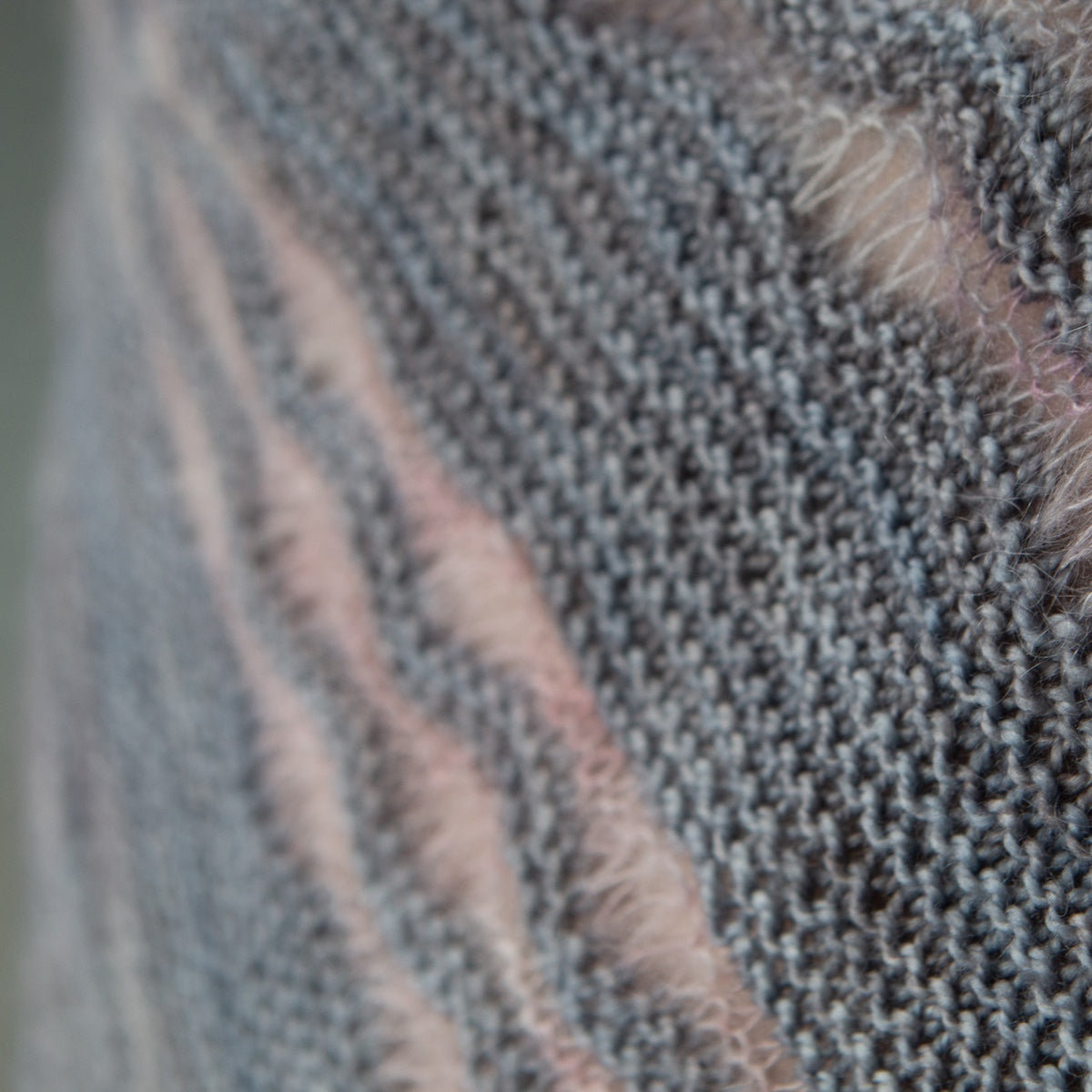This is a detailed close-up photo of an intricate arrangement on a reddish-brown surface, possibly fabric or netting, featuring 20-25 lines of gray material that could be yarn, chains, or some type of rope. The gray lines are placed side-by-side in somewhat wavy, non-parallel rows, and while the upper right portion of the image is sharply focused, the left side is blurry. The arrangement forms a square-like pattern and the gray material varies in thickness, with some sections appearing densely packed and others more loosely arranged. The purpose of these lines is unclear; they might be part of an embroidered or knitted accessory, or they could be utilitarian chains used for holding or hanging items.